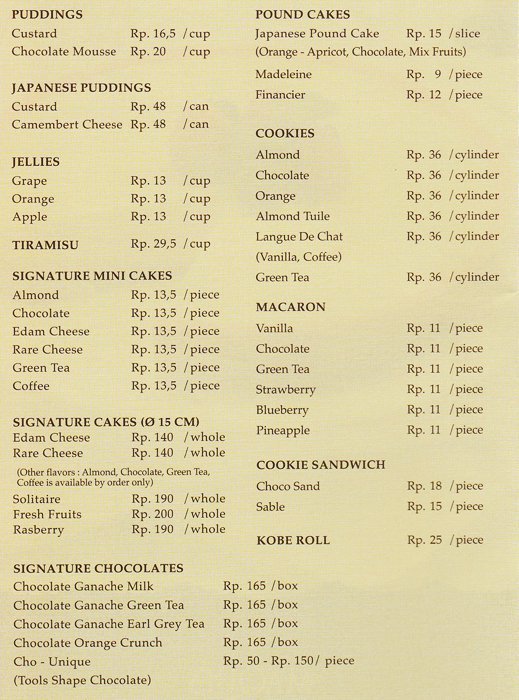The image depicts a rectangular menu card set against a light brown background with text in dark brown and black colors. The menu is organized into various categories, each with specific food items and their corresponding prices. The headings in dark black font include: puddings, Japanese puddings, jellies, signature mini cakes, signature cakes, signature chocolates, pound cakes, cookies, macarons, and cookie sandwiches. Under each heading, lighter black font lists the available items and their prices.

For example, under "Puddings," the menu offers custard and chocolate mousse, priced at rp.16,5 per cup. The "Japanese Puddings" section includes custard and Camembert cheese, also portioned by the cup or can. "Jellies" features flavors like grape, orange, and apple, priced similarly by the cup. There are also sections for tiramisu, various types of cakes such as edam cheese and fresh fruits, and chocolates including milk chocolate ganache and green tea ganache.

The menu continues with "Pound Cakes," followed by various "Cookies" such as almond cookies, each listed with their price and packaging type. For example, almond chocolate, orange almond tube, and Langue de Chat varieties have specified prices and content descriptions. The meticulous organization of the menu details the flavors, types, and prices for each category, making it clear and comprehensive for customers.